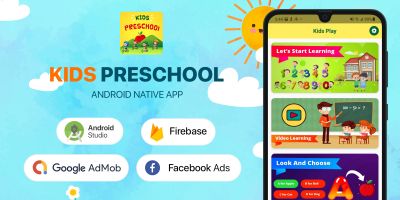This detailed image captures a small, cropped screenshot of a product description graphic for a children's app. The background features a whimsical, child-friendly design, portraying a cheerful blue sky dotted with puffy white clouds and a beaming sun with a smiley face. To the right of this vivid sky scene, there's a partially visible iPhone displaying the app's main screen prominently on its display.

Central to the image, towards the center-left, is a square thumbnail showcasing the app's logo, which is labeled "Kids Preschool." The text "KIDS PRESCHOOL" is spotlighted in large, capitalized letters, with "KIDS" in a vibrant orange hue and "PRESCHOOL" in a bold dark blue. Beneath this, the phrase "ANDROID NATIVE APP" is inscribed in small capital letters, centered neatly beneath the main logo.

Further down, two rows of small icons represent various associated apps and tools. On the bottom left, the Android Studio icon is positioned, while the Firebase icon is on the bottom right. Below these, the Google AdMob icon is placed on the left, and the Facebook Ads icon is on the right. The lower portion of the screenshot is cropped, leaving these elements as the main focus.